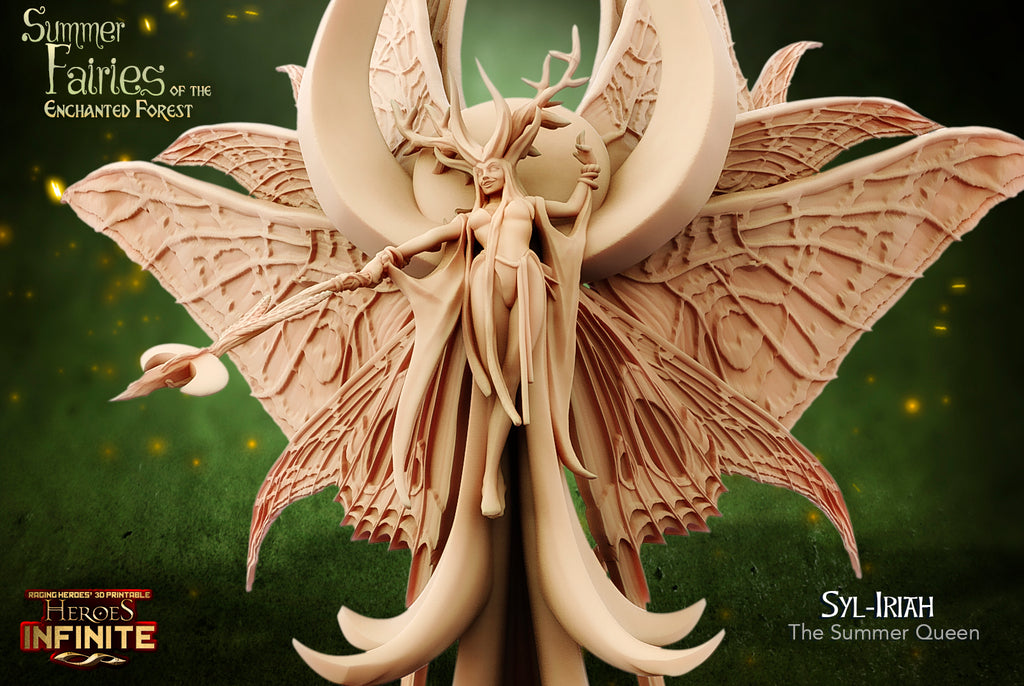The digital image, seemingly a 3D rendering of a sculpture, portrays a fantastical video game character named Syl Iria, the Summer Queen, part of the "Summer Fairies of the Enchanted Forest" collection. Dominating the frame is a majestic goddess-like figure crafted to simulate an ivory or light tan material. Syl Iria is depicted with voluminous hair and prominent antlers. She has multiple large, butterfly-like wings – potentially six or more –, each veined like those of a reptile, arranged in pairs with the tips of some just visible at the rear. Below her, a tail formed in the style of swallowtail butterfly wings extends down. She stands above a circular mandala pattern of curved tusks nearly matching her in size.

Syl Iria is dressed in a form-fitting outfit that resembles a bathing suit and is accompanied by flowing fabric. She wields a bladed weapon or baton in her right hand, positioned downwards and to the left. Surrounding her shoulders and cresting above her head are circular arrangements of tusks or horns. The backdrop is a blurred and grainy green scene with light particles akin to fireflies, evoking a verdant forest atmosphere. The top left corner of the image contains the title "Summer Fairies of the Enchanted Forest," while the bottom left features the label "Heroes Infinite Raging Heroes 3D Printable" and the character's name, "Syl Iria, the Summer Queen," in the bottom right.